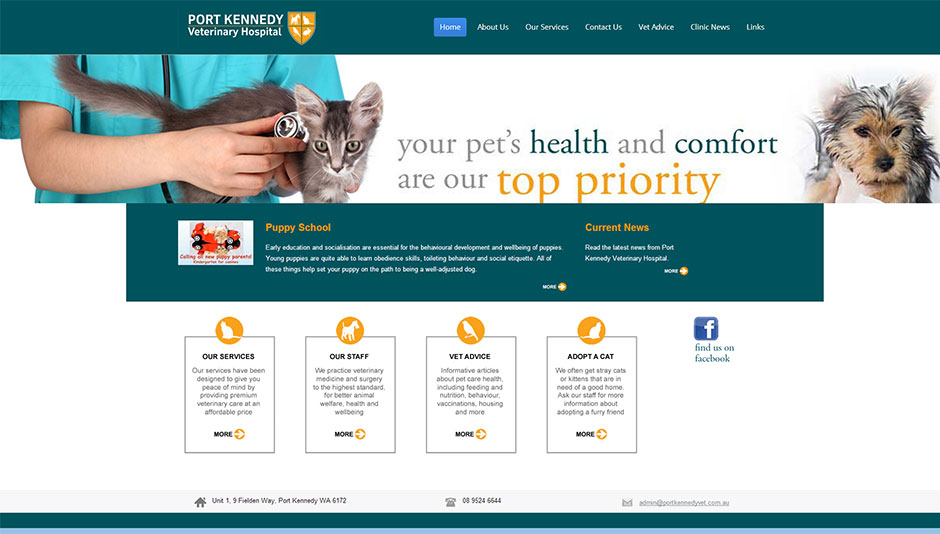This screenshot appears to be from the website of the Port Kennedy Veterinary Hospital. At the top of the page, there's a dark green banner that reads "Port Kennedy Veterinary Hospital." To its right, there's a yellow shield divided into four sections, each featuring a silhouette of a different white animal: a dog in the top left, a cat in the top right, a bird in the bottom left, and a rabbit in the bottom right.

To the right of the shield, there is a menu with headers including Home, About Us, Our Service, Contact Us, Vet Advice, Clinical News, and Links. Below the banner, on the left side, there's a picture of a veterinarian wearing an aqua green short-sleeved smock, gently holding a grayish cat with white spots on its mouth and chest. The cat also has large ears and striking green eyes, and the veterinarian is using a stethoscope on its neck. The veterinarian is shown from the torso up in this image.

Centered on the page is the message: "Your pet's health and comfort are our top priority." To the right of this message, there's an image of a wet dog with gray fur and a brown face.

Below this section, there's a green text box containing more information, including sections titled "Puppy School" to the left and "Current News" to the right. Further down, there are various informational boxes labeled Our Services, Our Staff, Vet Advice, and Adopt a Cat. Each box has an icon in a yellow circle: a cat for Our Services, a dog for Our Staff, a bird for Vet Advice, and another cat for Adopt a Cat. There's also a Facebook icon to the far right, indicating the hospital's social media presence.